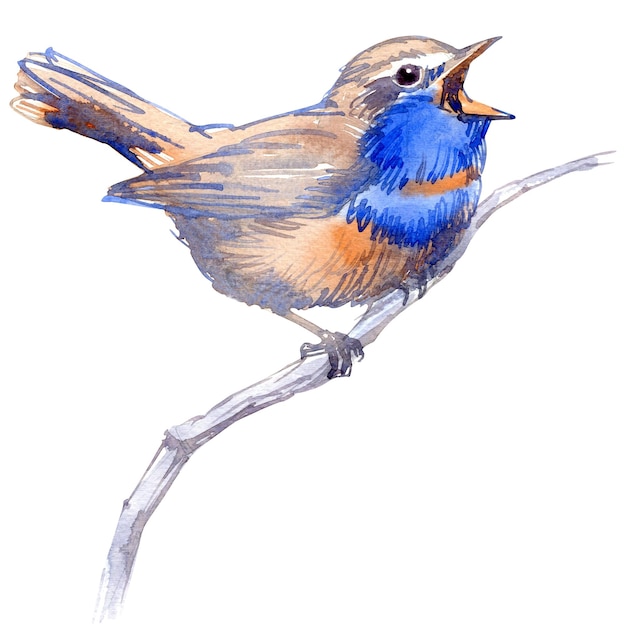The image is a detailed, illustrative sketch of a bird perched on a thin branch set against a solid white background. The branch extends diagonally from the upper right to the lower left, rendered in light gray with darker brown lines for texture. The bird faces right with its beak wide open, appearing as though it's singing. Its beak is orange and prominent on the right side of the composition. The bird's body displays a mix of vibrant and subtle hues: the underside is predominantly blue with interspersed streaks of orange and brown. The head features a large, black eye with a white stripe above it, surrounded by medium and light brown feathers. The wings and tail also exhibit similar shades of brown, complemented by a blue outline tracing the bird's silhouette. The legs and claws grasping the branch are brown and thin. The bird’s overall rounded form, small size, and varied coloring give it a lively and expressive presence on the minimalist backdrop.